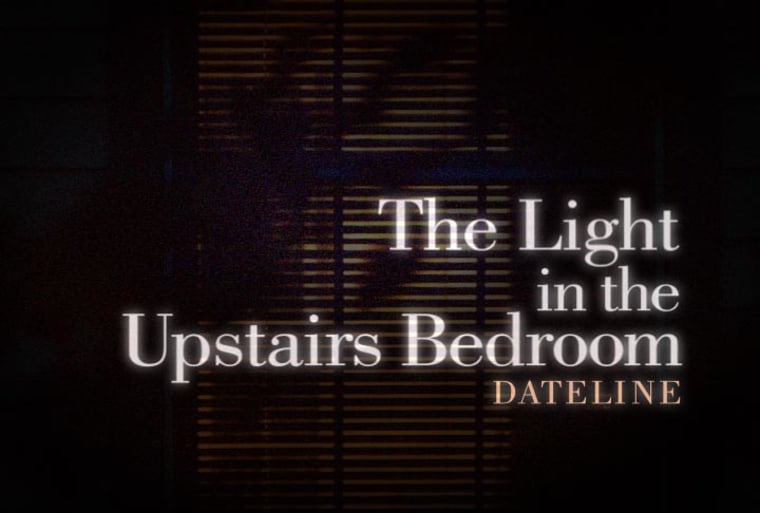The image depicts a dark scene with a nearly black background, creating a mysterious and somewhat eerie atmosphere. It appears to show window blinds, mostly in black, with two vertical lines running downward, hinting at the structure of the blinds. There is a faint bluish reflection at the top, adding to the obscurity. The centerpiece of the image is text in a glowing font format: the phrase "The light in the upstairs bedroom" is written in a white serif font and is indented to the right. Below it, "DATELINE" appears in a yellow, serif font and is also aligned to the right, though the phrase "the upstairs bedroom" is centered. The overall impression is one of darkness with elusive elements highlighted by the unsettlingly specific text, highlighting the light in an otherwise shadowy scene.